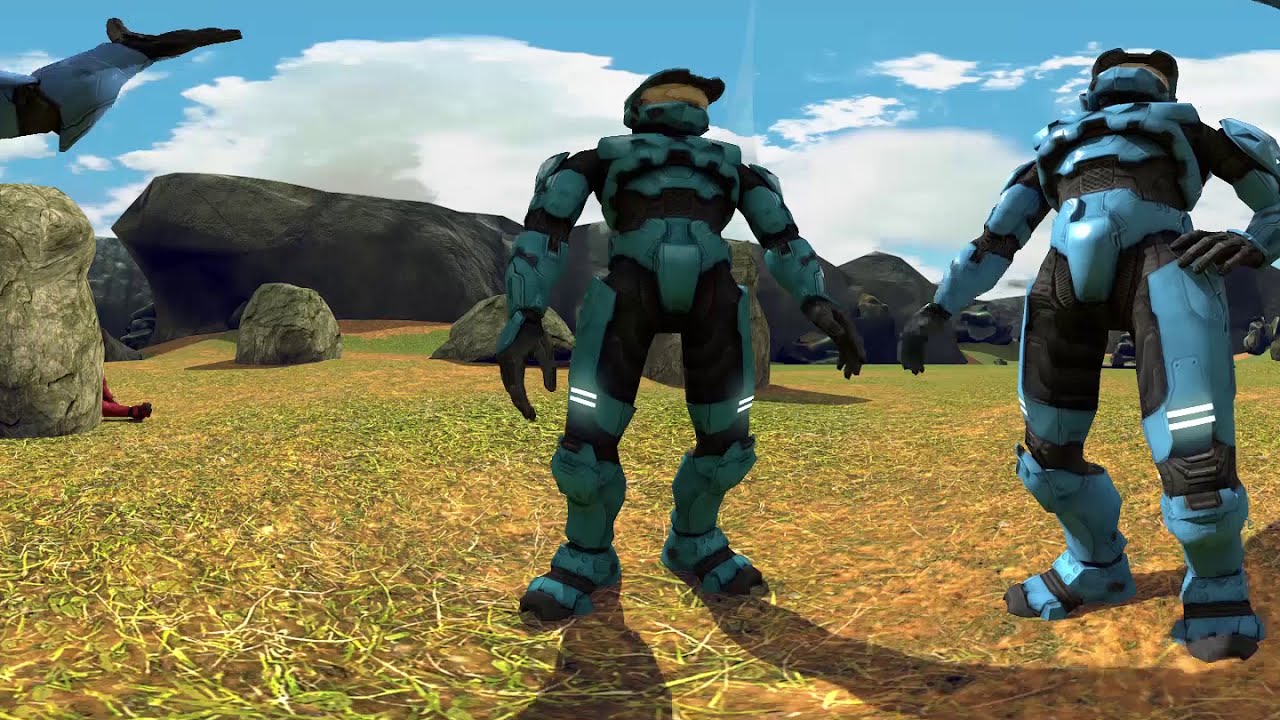This detailed image appears to be a computer-generated screenshot, likely from the video game "Halo". The scene showcases three characters donned in high-tech exoskeleton armor, characteristic of Halo's Spartans. Each character wears a full helmet with gold visors and body armor predominantly in shades of blue and black, accented with glowing white lights on the knees and other segments of their gear. The characters are posed on a grassy, clay-like field interspersed with rocks, under a bright sky dotted with clouds. In the background, futuristic vehicles resembling jeeps add to the sci-fi atmosphere. One character stands with hands on hips, another in a neutral stance, and a third barely visible, making a gesture with their hand. The image has a slight panoramic distortion, enhancing a 360-degree effect.